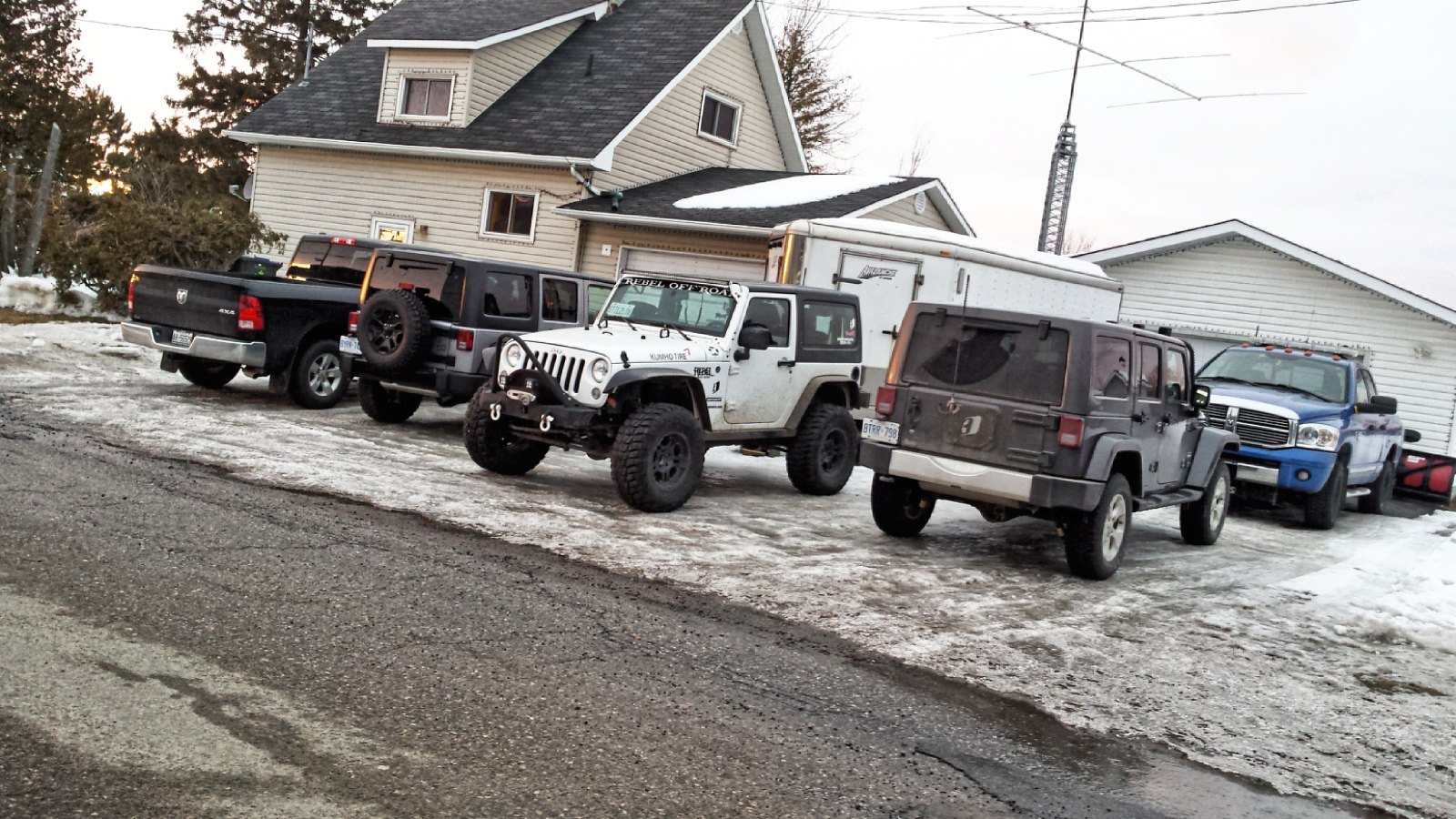This image, seemingly captured in a wintry or snowy region, features a cold, snow-covered setting. At the center is a two-story house with beige siding and a gray roof, showcasing an attached single-car garage and a detached garage. In the foreground, a snow-covered parking area on the right side of the image contains five vehicles, including three Jeeps—two Jeep Wranglers and a boxy Jeep vehicle—and two Dodge trucks, one black and one blue. Additionally, a white trailer is attached to one of the Jeeps. Along the road, which runs from the bottom right to the middle left of the image and appears clear of snow, likely due to traffic, the vehicles are meticulously parked. Snow blankets the ground around the house, and towards the top right, a large antenna rises against the white sky, while trees occupy the top left corner.